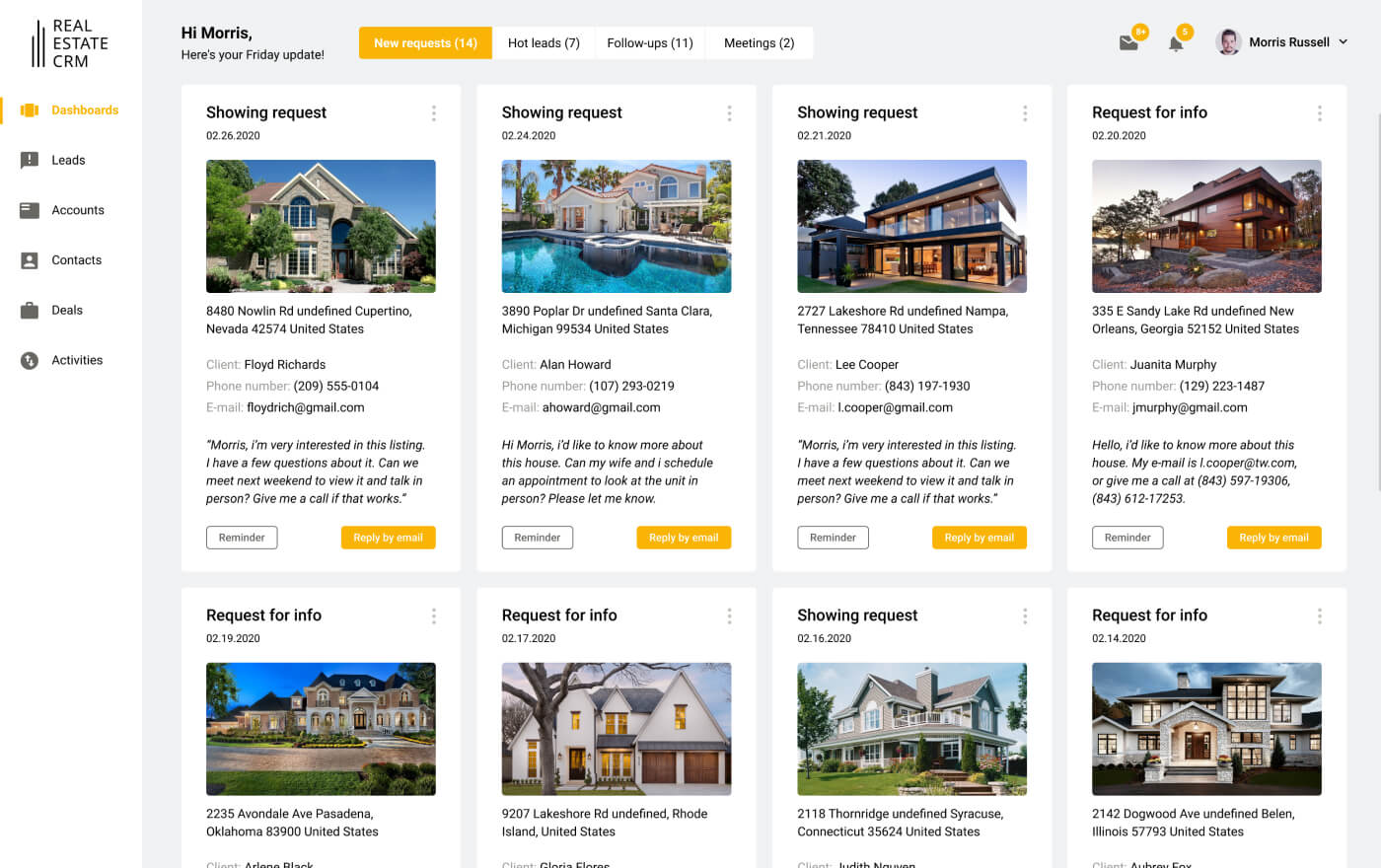The image displays a real estate Customer Relationship Management (CRM) interface. In the top left corner, the CRM logo is visible. Down the left side of the interface, there is a vertical menu with options listed in black text, including Dashboard, Leads, Account, Contacts, Deals, and Activities. The Dashboard option is currently highlighted in orange.

The main screen greets the user with "Hi Morris," followed by the "Friday Update," which includes key statistics: 14 new requests, 7 hot leads, 11 follow-ups, 2 meetings, and 2 showing requests.

Detailed client interactions are displayed below. For instance:

1. A request dated 26th February 2020, involves a property at 8480 Nowlin Road, Caperito, Nevada, 42574, United States. The client, Floyd Richards, has reached out via phone (209-555-0104) and email (floydrich@gmail.com), expressing interest in the listing and requesting a meeting next weekend to discuss it in person. A reminder prompts Morris to reply to this email.

2. Another request, dated 24th February 2020, details a showing at 3890 Popular Drive, Santa Clara, Michigan, 99534, United States. The client, Allen Howard, has contacted through phone (107-293-0219) and email (ahoward@gmail.com), initiating the conversation with "Hi Morris."

The interface encapsulates critical updates and client engagements, imperative for Morris’s real estate dealings.